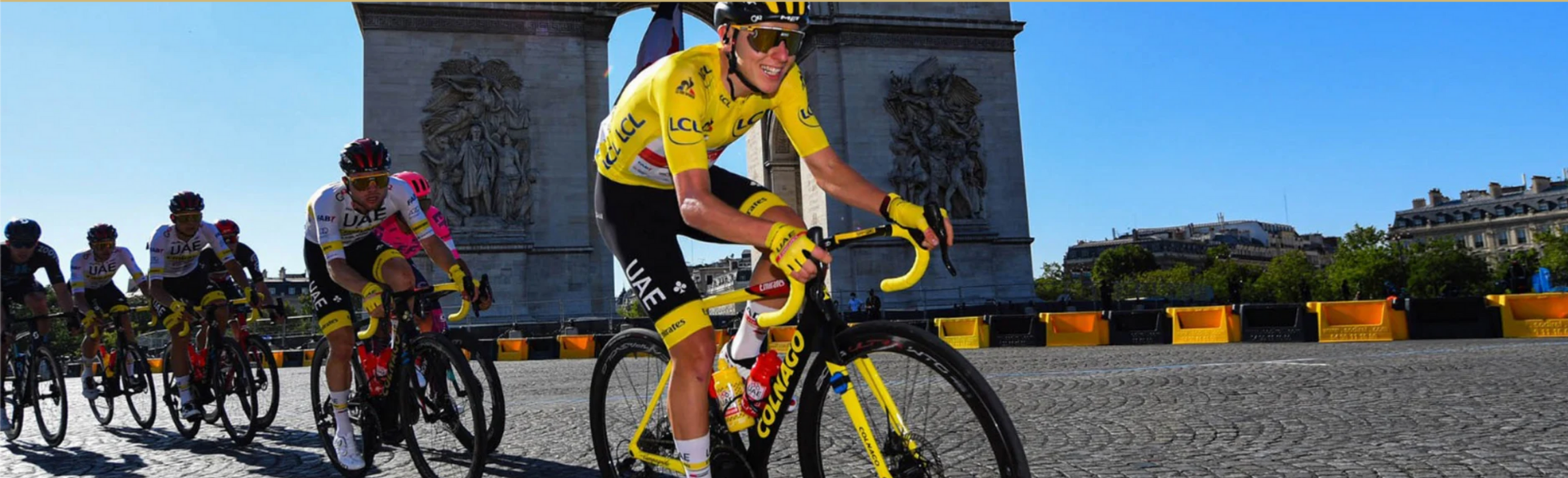This panoramic image captures a vibrant scene of a cycling race, possibly the Tour de France, taking place in Paris. The focal point of the image is the iconic Arc de Triomphe prominently displayed in the background, signifying the race's location. The sky is a brilliant blue with no clouds, suggesting a perfect sunny day. Leading the pack of around eight cyclists is a rider in a striking yellow and black uniform, complete with a matching helmet and a bike branded Colnago. The leader, who also sports reflective sunglasses, has the initials "UAE" on his shorts, indicating his team, the United Arab Emirates. Behind him, other cyclists can be seen in various uniforms: one in hot pink and black, another in black with an orange helmet, and one entirely in black. The area around the race is clear of spectators, although there might be some figures obscured behind barriers. The cyclists move energetically through the street, with European architecture providing a picturesque backdrop.